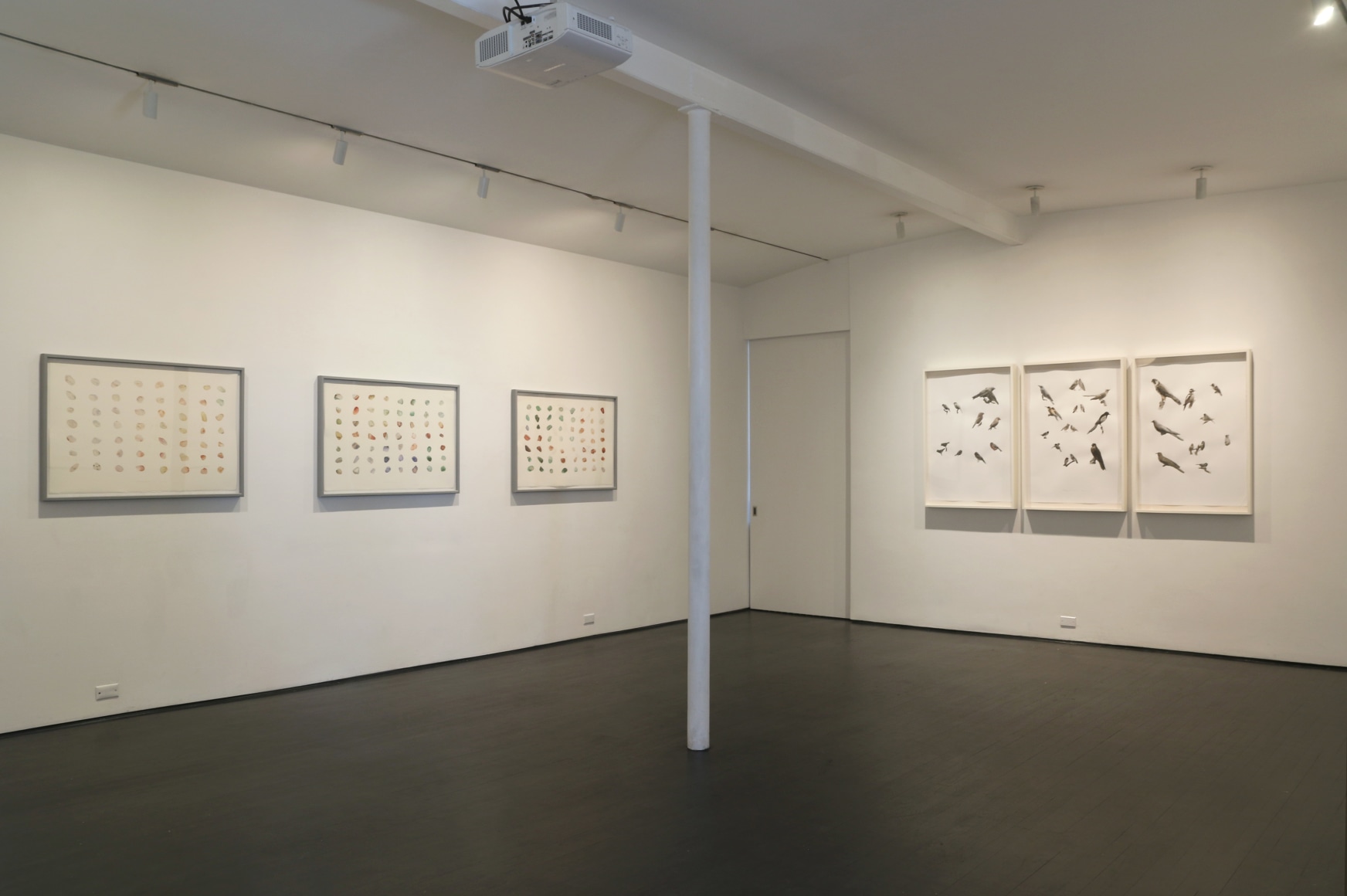The image depicts the interior of an art gallery with a stark and minimalist design. The gallery space boasts pristine white walls and ceilings, contrasted by dark wooden floors. A slim, unadorned white support column stands in the middle of the room, supporting a ceiling beam. Track lighting, equipped with adjustable can heads, illuminates the space. On the ceiling, there's a garage door-like contraption that may serve as an air conditioning or filtration system.

Artwork adorns the gallery walls, with two sets of framed illustrations. On the right wall, three paintings feature various types of birds, presented in a collage style without any accompanying text. Each painting showcases multiple birds, intricately detailed in white frames mounted on the white wall. The left wall also displays three framed prints, possibly of butterflies, adding a hint of color with subtle reds and blues speckled throughout the images.

At the far end of the room, a door stands slightly ajar in the back corner, maintaining the understated aesthetic. Enhancing the presentation of the artwork, a large projector-type light hangs from the ceiling, casting focused illumination on the paintings. The overall ambiance of the gallery is serene, with a harmonious blend of cream, white, and soft hues.